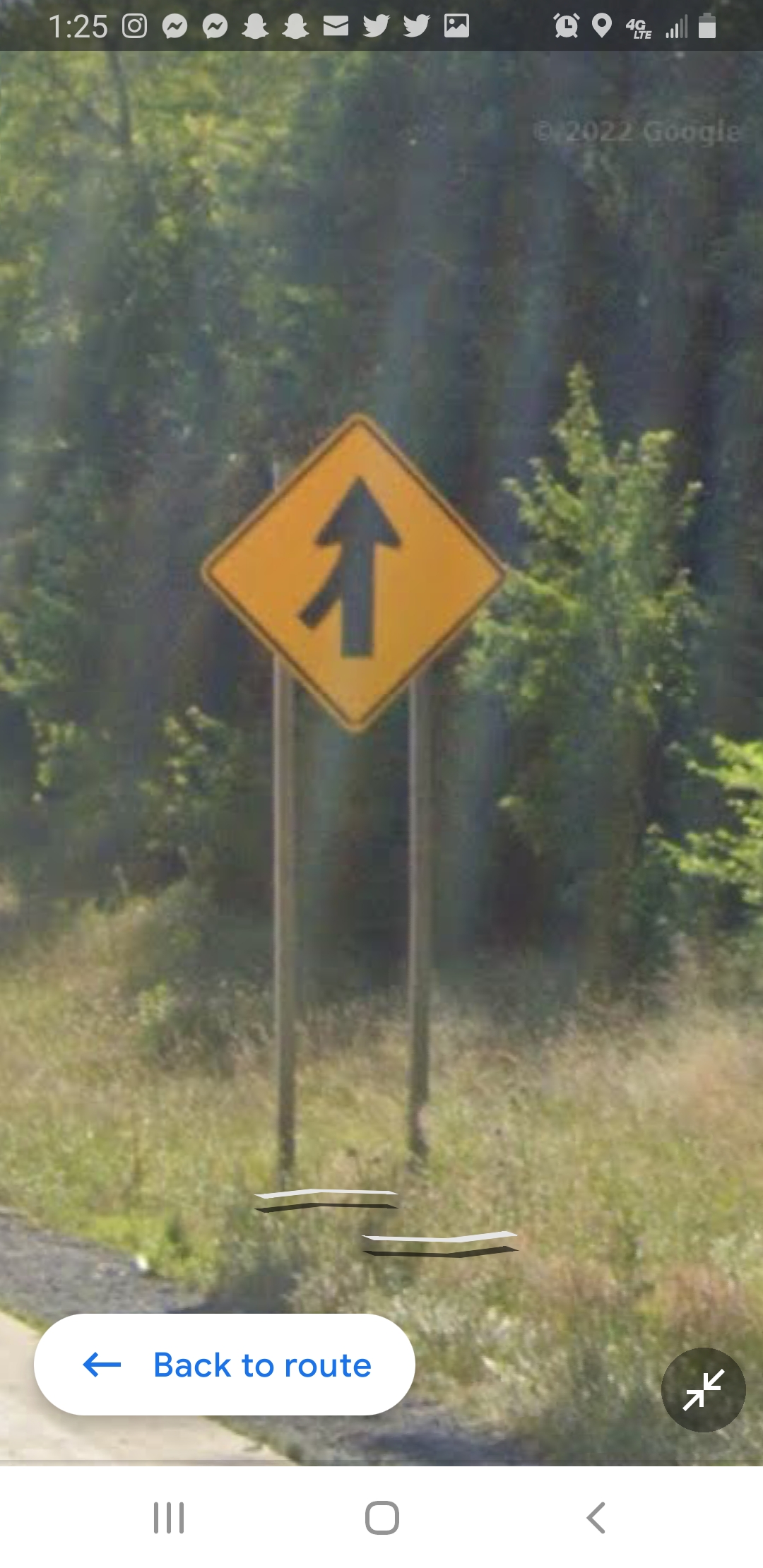The image, a screenshot likely taken from a smartphone, showcases an outdoor scene featuring a yellow, diamond-shaped traffic sign mounted on two metal poles. The sign displays an arrow pointing straight up with a merging line coming in from the left, indicative of an upcoming merge on the roadway. Surrounding the sign are lush green trees and grass, creating a verdant backdrop. The ground below the sign transitions from gravel to pavement. In the lower part of the image, there is a white bubble or banner reading “Back to route” with a blue arrow pointing to the left, suggesting a navigational option. The top edge of the screenshot displays typical smartphone icons and white numbers, while the bottom right corner features a darkened circular area with two diagonal arrows pointing towards each other. The upper right corner contains a faint watermark noting “© 2022 Google.” The overall brightness and clarity suggest a sunny day, casting a slightly overexposed light across the scene.